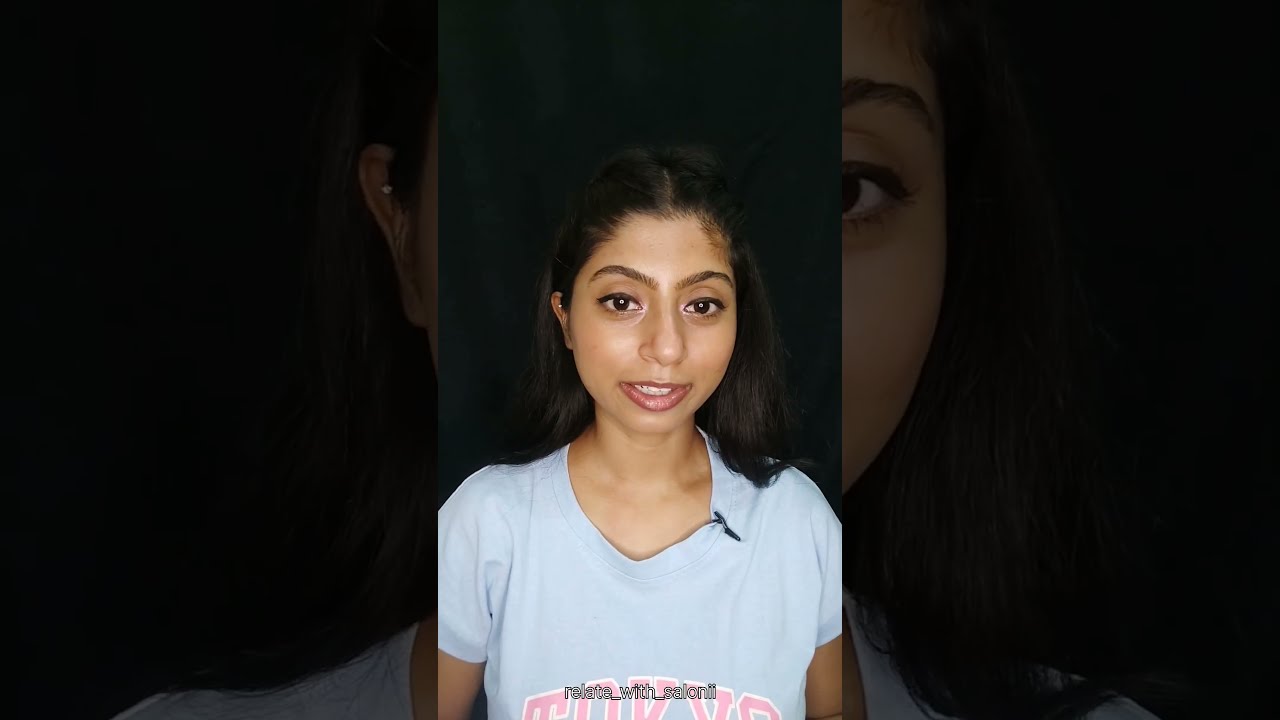The image is a vertical cell phone-style portrait of a woman against a black background. The central image shows the woman from her upper chest to the top of her head, with a zoomed-in, faded version of the same image used as the background. The woman has dark shoulder-length hair parted down the middle and brown skin. She is facing the camera with a slight smile or smirk, about three feet away. She is wearing a light blue t-shirt with a graphic on the chest that reads "Tokyo" in pink text with a white border. A microphone is clipped to the left side of her shirt collar. Additional features include her red lipstick, large eyebrows, and brown eyes. There is also some white text superimposed on the image, which appears to be the name of the photo, consisting of three words separated by underscores.